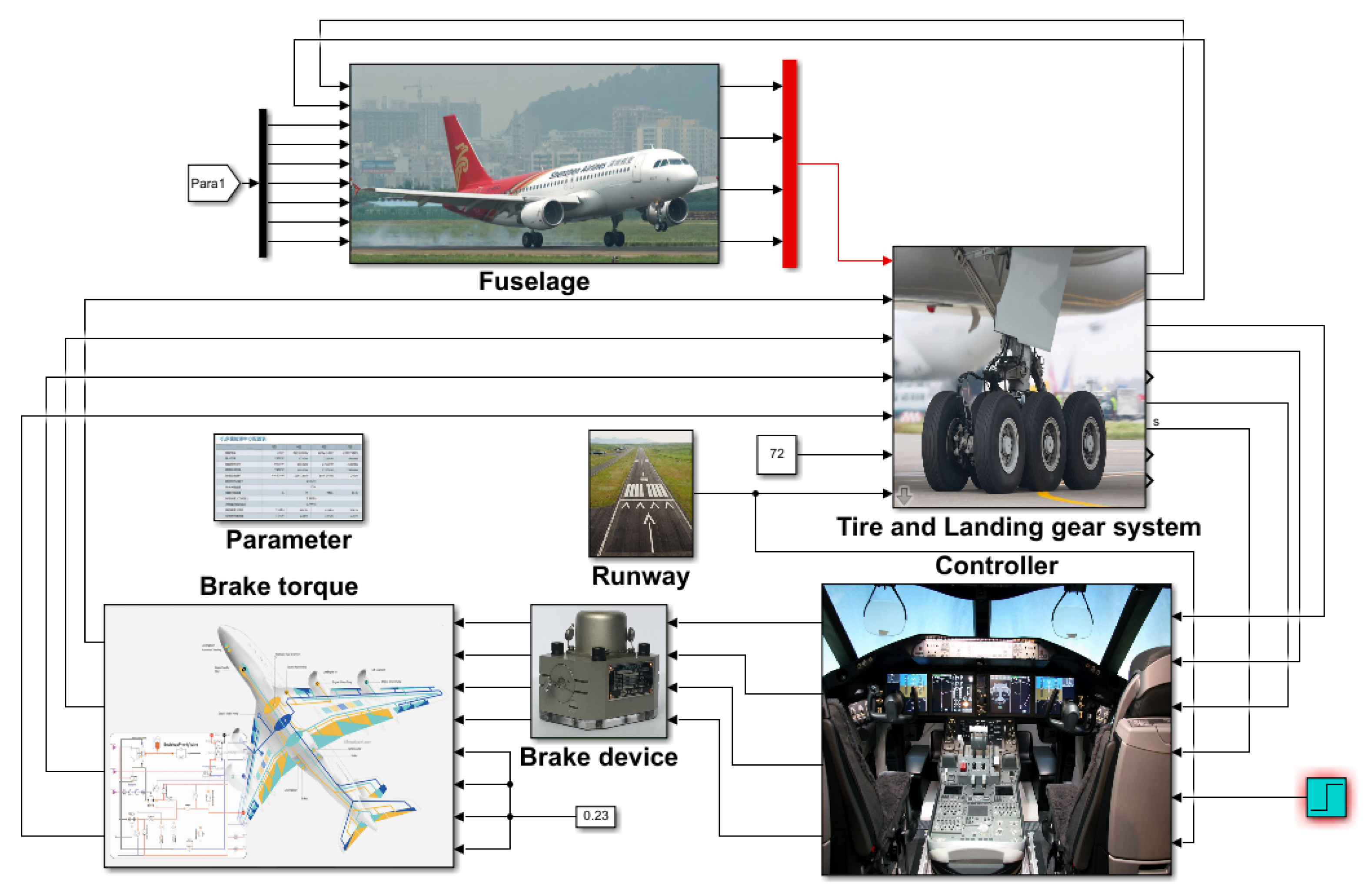The image is a detailed diagram of a jet plane with a sleek silver front and a vibrant red tail. Although the company's logo is not discernible, the diagram is meticulously annotated with numerous arrows pointing to various sections of the plane, each accompanied by corresponding images and descriptions. At the top of the diagram, annotations highlight the fuselage of the aircraft. Diagonally to the right, there is a focus on the tire and landing gear system. In the center of the image, labels denote the parameters and runway specifications. The bottom section elaborates on the brake system, featuring a detailed but small diagram that remains unclear. Additionally, it mentions the brake torque and a controller, which appears to represent the cockpit. Overall, this diagram serves as an informative guide to the multiple components and mechanisms of the jet plane.